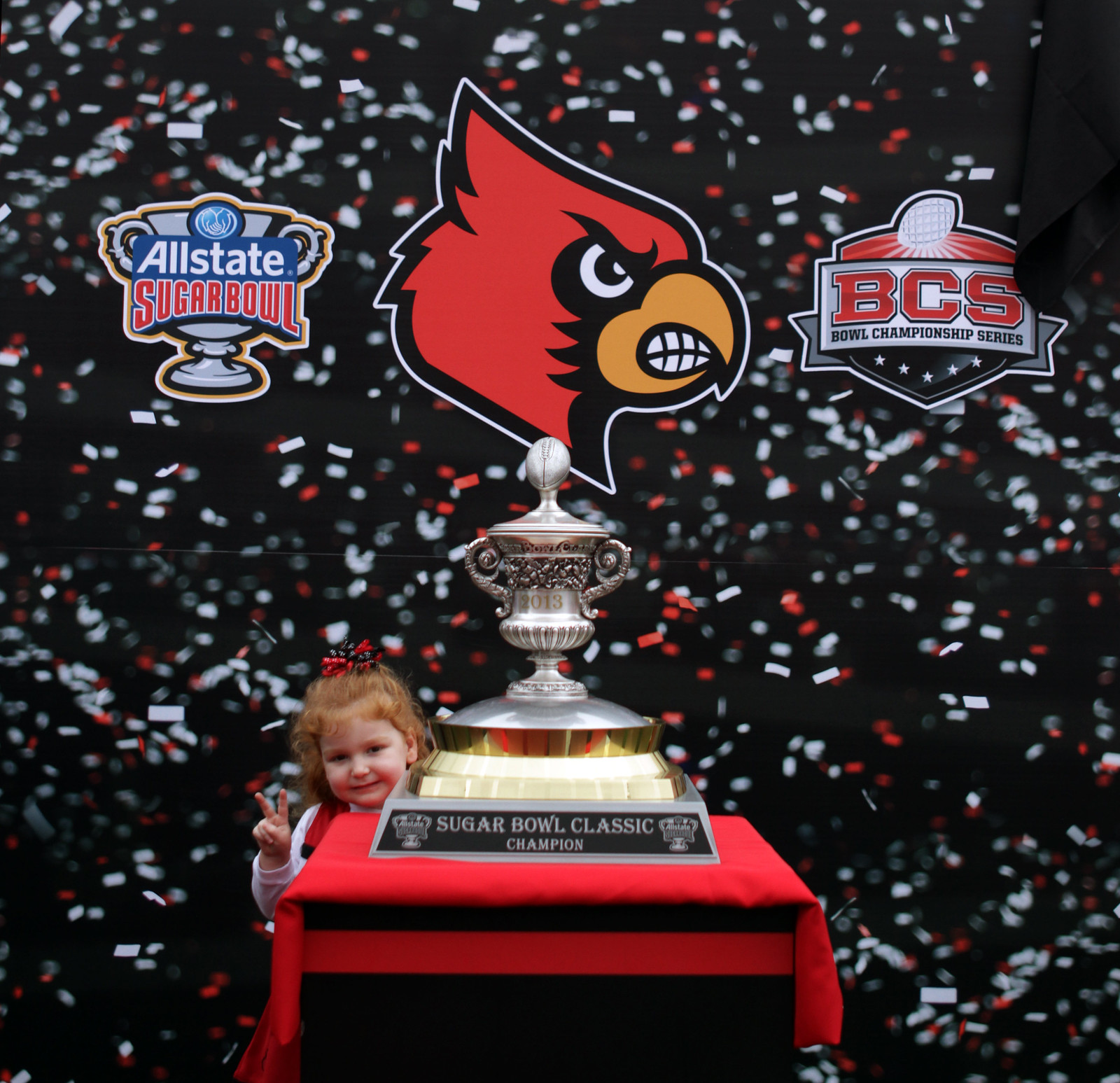This color photograph depicts a celebratory scene likely from a sporting event. At the center is a red pedestal supporting a large, silver, chalice-shaped trophy with a plaque reading "Sugar Bowl Classic Champion." The pedestal boasts two smaller trophies on either side of the plaque. The backdrop is a solid black field filled with red and white falling confetti.

To the left of the pedestal stands a young red-haired girl, adorned with a red bow, casually dressed in a red top with white sleeves. She is joyfully holding up a peace sign with her right hand. Above the trophy, three prominent logos are overlaid: on the left is an emblem reading "Allstate Sugar Bowl" accompanied by a trophy graphic, in the middle is the logo of a cardinal head featuring red plumage, a black mask, and an angrily exposed yellow beak, and to the right is the "BCS Bowl Championship Series" logo in red and grey.